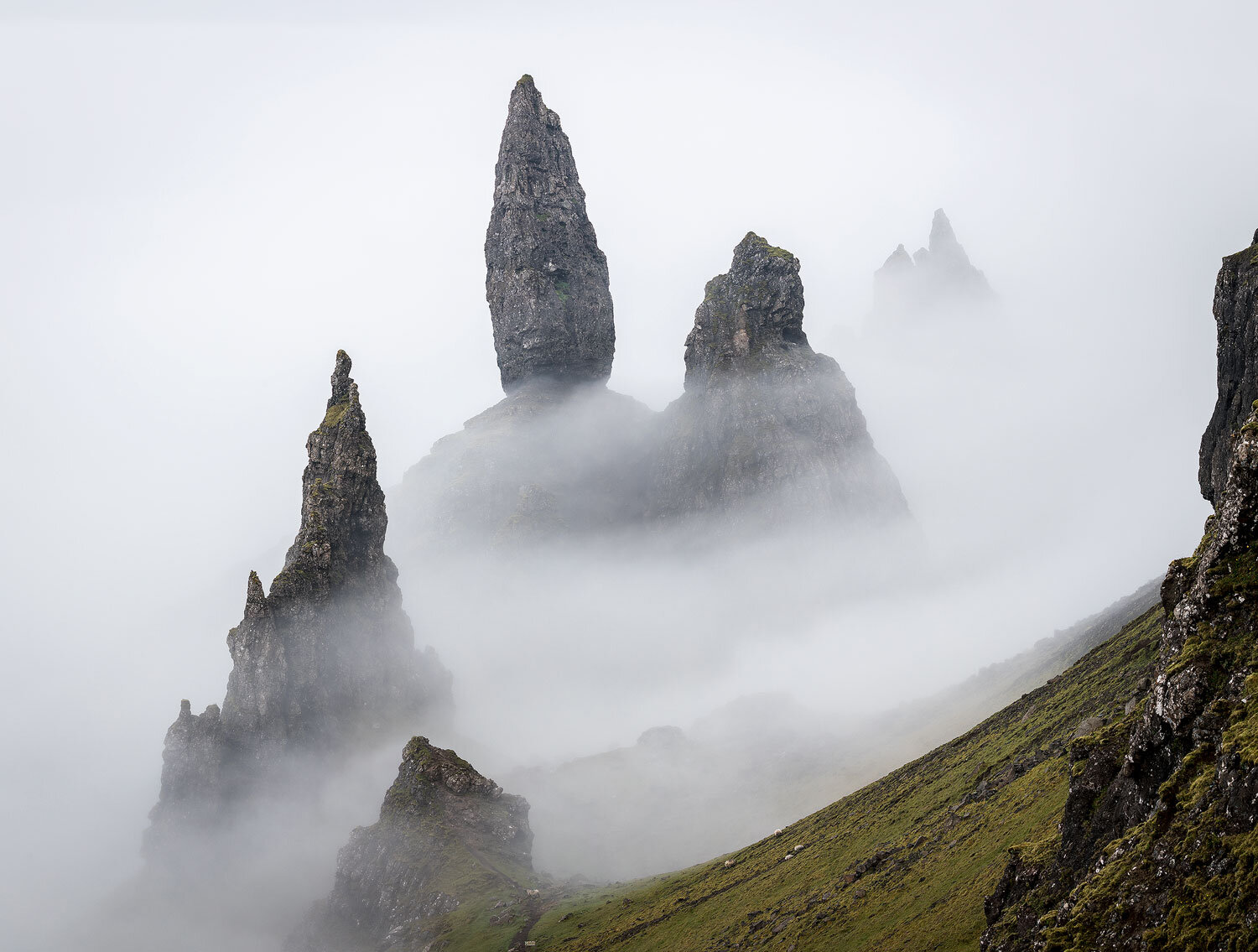This color photograph, likely enhanced with Photoshop effects, captures a dramatic outdoor landscape in a high mountain valley. The image is oriented in landscape format and features a foreground with a gently sloping hillside, covered in greenish moss and dotted with dark gray and brownish-black rocks. In the bottom-left corner, a prominent pointed boulder stands near a triangular-shaped rock with multiple peaks, reaching upwards like natural monuments sculpted by time. The hillside continues from the top right with a rocky outcropping partially cut off on the right edge, transitioning into another steep cliff.

Dominating the scene, a thick, airy fog envelops the valley, moving in from the upper left corner and obscuring the finer details of the background. The fog is so dense in places that it blurs the outline of features, revealing only their ghostly silhouettes. On the right-hand side, some green low plant life is visible underneath the rocky cliffs. High above, an imposing double-peaked mountain stands tall against the mist, adding to the mystique of this rugged and natural landscape. The soft blue sky at the top left fades into this mist, enhancing the ethereal atmosphere of the scene.